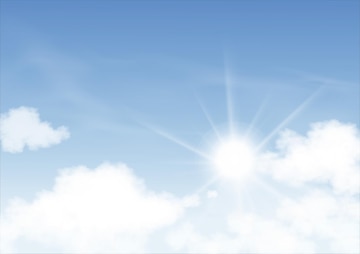The image depicts a vibrant sky transitioning from a deep blue at the top to a lighter blue as it approaches the horizon. The sun, positioned slightly above the midline and about two-thirds from the left, radiates a brilliant white light. Its intense luminosity creates a distinct starburst pattern, with rays spreading out in all directions—up, down, left, right, and at various angles. These rays add dynamic energy to the scene, although the sun's brilliance obscures finer details near its center. The bottom and bottom right of the image are graced with pure white, fluffy clouds, while a solitary puffy cloud can also be found around the left-center area. Above these clouds, the sky remains mostly clear, with only faint wisps or a slight haze interrupting the azure expanse.